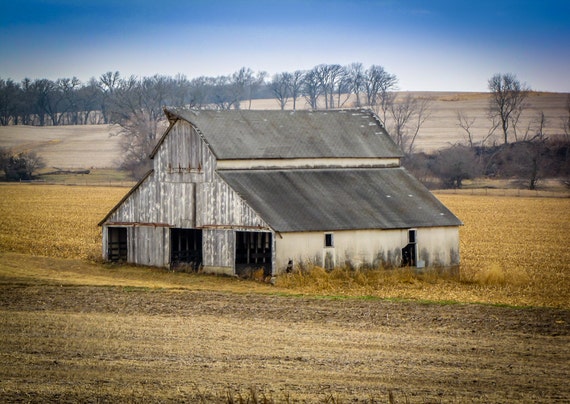This image showcases an expansive outdoor landscape centered around a large, old gray barn with three sizable doors on its wooden facade. The barn, which also features sections of white and gray planks and two small windows on the right, is crowned by a gray roof. It sits prominently in the middle of a vast, yellowish field, suggesting dried grass or crops, typical of a fall setting. The foreground of the image presents a mix of brown and lighter gray dirt, extending across the entire scene. Surrounding the barn, there are trees without leaves, varying from rows to the left to sporadic placements on the right, all contributing to the autumnal atmosphere. In the distance, rolling hills also bare without leaves enhance the sense of a serene fall day under a sky that transitions from blue at the top to white towards the middle.